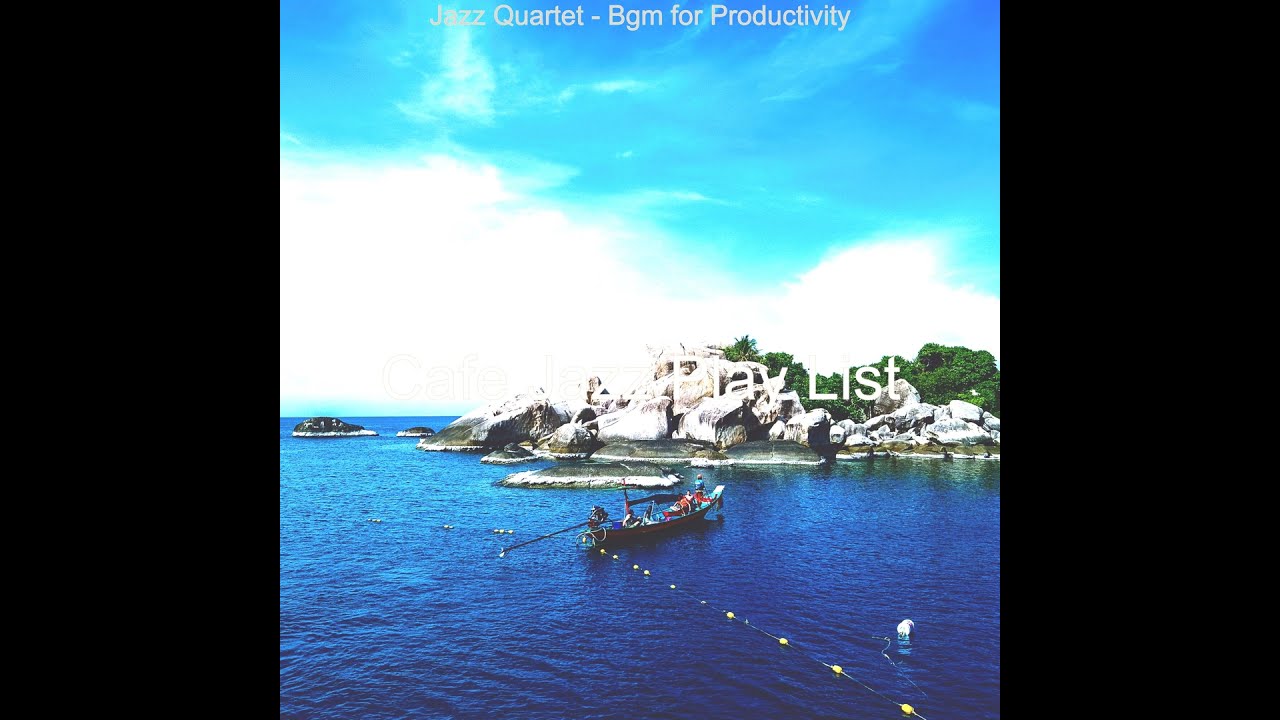The photograph depicts a tranquil, sunny scene of a rocky island surrounded by calm, dark blue water. The island, featuring large gray stones, has green trees growing atop it, providing a sense of rugged natural beauty. Above, the sky is a clear blue with wispy clouds and some denser clouds in the distance.

In the foreground, a long, narrow boat, possibly a fishing or tourist boat with wooden components and a small mast, floats serenely on the water. The boat is centered in the image and is accompanied by a yellow fishing net or buoy line that stretches from the right-hand corner towards the center-left, adorned with yellow buoys.

Text at the top of the image reads: "jazz quartet BGM for productivity." However, parts of the text are obscured by white clouds, and the word "playlist" is partially visible in the center, though some letters are difficult to discern against the bright background. The overall setting is outdoors, captured as if from the perspective of someone on the water, emphasizing a serene and picturesque maritime environment.